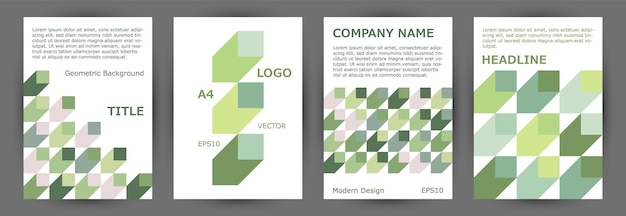This image is a horizontally aligned rectangular poster with a medium to dark gray background, showcasing four vertical white pages side by side, each detailing elements of a graphic design layout. Starting from the left, the first page features a light gray left-aligned paragraph at the top, followed by the text "geometric background" in smaller black font, and "TITLE" in bold, all-caps green letters. The lower portion is adorned with a cluster of three-dimensional cubes in varying shades of green, light green, dark green, gray, white, and light blue, seemingly projecting outward.

The second page prominently displays three three-dimensional rectangular shapes aligned vertically. Adjacent to these shapes are designations in green, with "LOGO" in all-caps and "A4" labeled below, followed by "vector" and "EPS-10."

Moving to the third page, "COMPANY NAME" is prominently written at the top in all-caps green. Below it, there's a left-aligned paragraph, and the lower section showcases a similar assembly of three-dimensional rectangular shapes in different shades of green and related colors, accompanied by the text "modern design" and "EPS-10."

Lastly, the fourth page has a top section featuring roughly four lines of left-aligned text above the title "HEADLINE" in all-caps green. Below this headline are nine larger three-dimensional cubes in shades of green and related colors, also arranged to appear as if extending towards the viewer.

The cohesive elements like the geometric, cube-oriented visuals and the consistent use of green and gray accents tie these pages together, suggesting they belong to a unified branding or graphic design presentation.